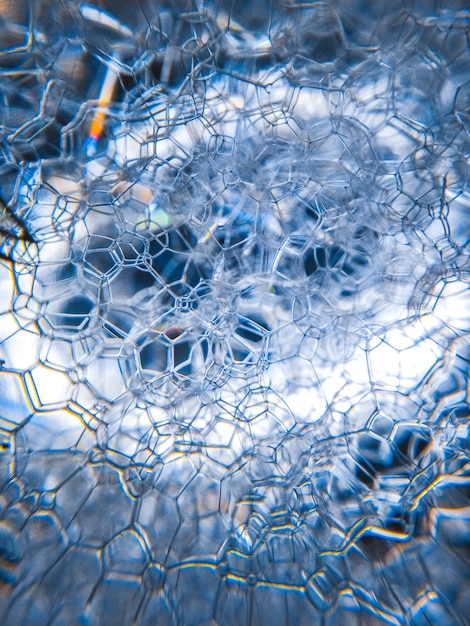This macro-style photograph captures an intricate and mesmerizing display of interconnected, angular soap bubbles. The bubbles create a complex, almost spiderweb-like pattern, with thin, blue lines outlining their edges. The arrangement appears multi-layered, giving a sense of depth and intertwined structure, akin to multiple chain link fences overlapping. The color palette is primarily blue, with glossy white highlights glistening on the bubble surfaces, contributing to the translucent and reflective characteristics typical of bubbles. In the top left corner, a soft, rainbow-colored glare is visible, reminiscent of light refracting through soap bubbles. Through the layers of bubbles, a blurry white ring with a darker center can be seen in the background, adding to the dreamlike quality of the image.